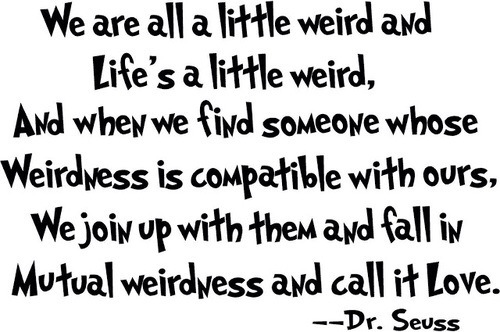This is a black and white digital image consisting solely of text on a completely white background. The text is presented in a playful, cutesy font reminiscent of Dr. Seuss's style, fitting for the quote attributed to him. The quote reads: "We are all a little weird, and life's a little weird. And when we find someone whose weirdness is compatible with ours, we join up with them and fall in mutual weirdness and call it love." The formatting is unique with certain letters randomly capitalized; every line break starts with a capital letter, even mid-sentence, and the word "Love" has its first letter capitalized. The text is black and bold, standing out clearly against the plain white background, with "Dr. Seuss" appearing in a slightly smaller font at the bottom right.